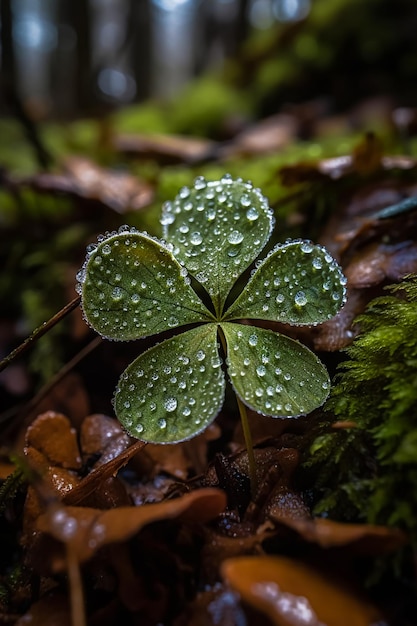A delicate five-petaled clover emerges from the wet forest floor, with each petal being light brown at the top and adorned with perfectly clear, circular droplets of water, suggesting recent rain. The clover's slender stem stands amidst a ground scattered with many brown leaves in the foreground and some green leaves to the right. Beyond the plant, the background blurs into an array of vague vertical black tree trunks, patches of greenery, and light filtering through the forest, creating a serene and tranquil daytime scene. The focus on the clover and its water droplets contrasts sharply with the soft, out-of-focus forest behind, emphasizing the intricate beauty of the tiny plant.